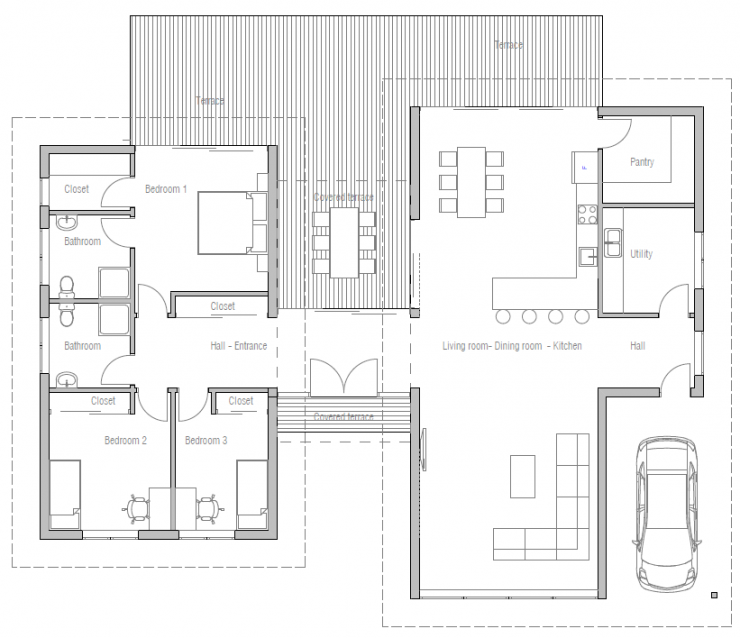The image is an overhead, black-and-white blueprint showcasing the detailed floor plan of a single-story home. The layout includes a designated parking area on the front right, leading to an entry door that opens into a hallway. This hallway connects to a utility room and then leads into the living room, dining room, and kitchen. Adjacent to the kitchen is a pantry. The blueprint also features both a main and additional covered terraces, one of which houses a long rectangular table. The plan meticulously outlines three bedrooms, each equipped with its own closet. Notably, there is a master bedroom with a private bathroom, alongside an additional shared bathroom. The entire schematic provides a comprehensive view of how different rooms and functional spaces are arranged throughout the house.